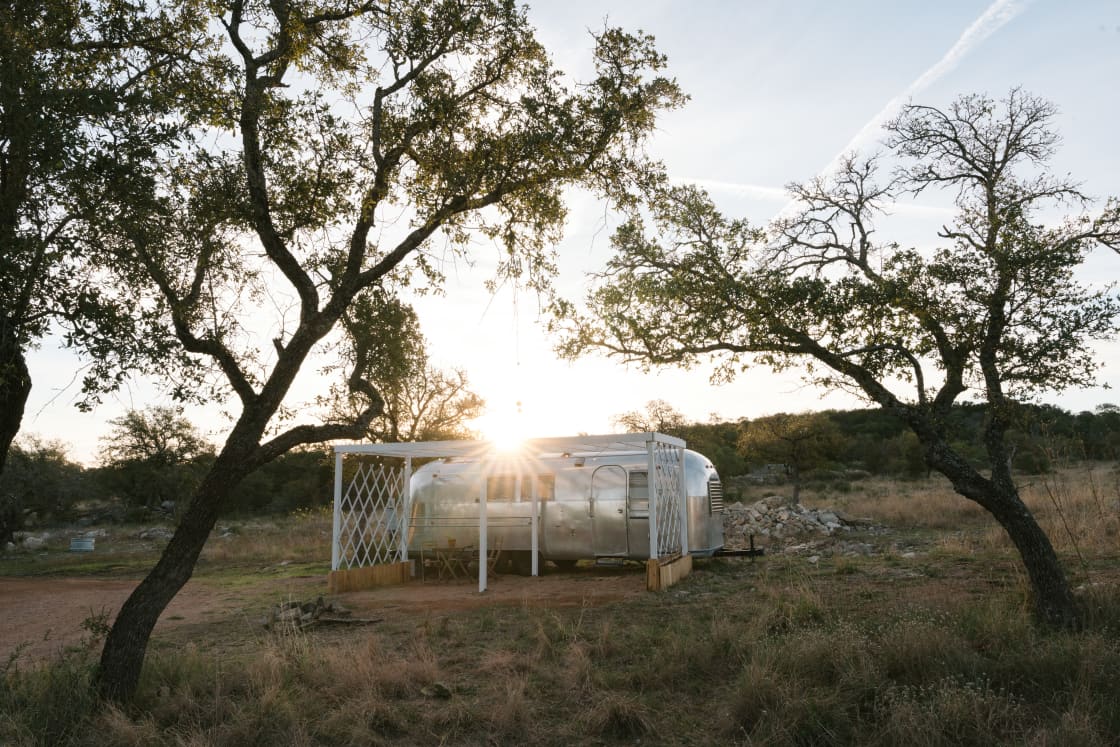This vibrant outdoor photograph, likely captured at sunrise, displays a serene, natural scene. The sky, a light pale blue with wispy clouds and contrails, meets the horizon, where the sun is just emerging from behind a tree-covered hill. In the foreground, the landscape is predominantly grassy with scattered areas resembling a field or plain, accented by wild vegetation.

Dominating the center of the image is a retro-style, shiny silver trailer, akin to an Airstream, boasting a well-preserved appearance. Attached to the trailer is a white trellis or arbor-like wooden structure, partially covered with lattice siding, suggesting a space for shelter or cooking. Despite the trailer's modern look, the surrounding area hints at past human activity with scattered objects like a large barrel possibly for watering livestock, charred remains indicating a possible fire pit, and a pile of rocks or concrete. 

Flanking the composition, two trees on the left and right frame the scene. The left tree enters the image diagonally, with several thick branches adorned with leaves, while the right tree, similarly angled inward, has fewer leaves, darkened by the overwhelming brightness of the rising sun. The entire setting conveys a feeling of quiet solitude, with no people present, enhancing the tranquil atmosphere of this early morning moment.